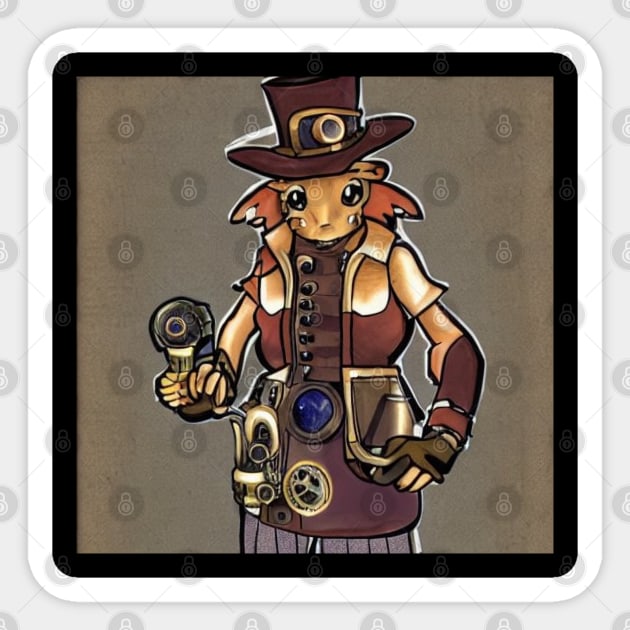The image depicts a locked character in a video game or a piece of private art, marked by a repeating combination lock-shaped watermark. The central artwork, encased within a gray background, white frame, and black outer frame, showcases a steampunk-style illustration of a humanoid creature of indeterminate origin. The creature, characterized by its large, wide-set dark eyes, protruding ears, and the notable absence of a visible mouth, sports vibrant red hair. It wears a tall brown top hat adorned with a brass spyglass device, and a sleeveless, western-style brown shirt. Draped over its torso is a leather apron festooned with typical steampunk tools, and each arm is fitted with a detailed gauntlet that partially covers its hands. This character bears an array of steampunk accessories—brass gears, funnels, pipes—visibly integrated into its gloves and apparel, accentuating the intricate, mechanical aesthetic.